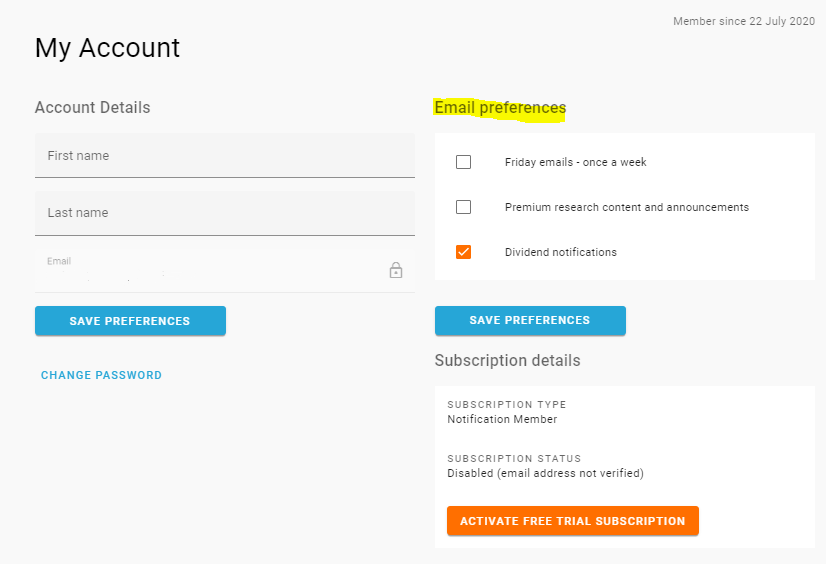The image is a screenshot of an account details page featuring a light gray background with text in various shades of black and gray. 

1. **Header Section**:
   - At the very top left of the image, "My Account" is prominently displayed in bold black lettering. 
   - The upper right-hand corner contains the text "Member since 22 July 2020".

2. **Main Body**:
   - Directly below the header is the label "Account Details".
   - Under "Account Details", in a dark gray rectangle, the following fields are listed sequentially:
     - "First Name"
     - "Last Name"
     - "Email" in a very light gray font accompanied by a small padlock icon indicating privacy or security.
   - On the right side of this section, highlighted with a yellow swoosh, is "Email Preferences".

3. **Email Preferences Section**:
   - Below "Email Preferences" are individual subscription options with corresponding checkboxes:
     - "Friday Emails - once a week" (unchecked box)
     - "Premium research content and announcements" (unchecked box)
     - "Dividend notifications" (checked box with an orange tick mark)
   - To the left under this section, there is a blue rectangular box labeled "SAVE PREFERENCES" in white font.
   - Further below is the option "CHANGE PASSWORD" in all caps and blue font. 

4. **Subscription Details Section**:
   - On the right side, below the "Email Preferences" section, another blue rectangular "SAVE PREFERENCES" box appears.
   - Beneath this is the "Subscription Details" header in darker font.
   - Under "Subscription Details", the following information is displayed:
     - "Subscription type: Notification member"
     - "Subscription status: Disabled (email address not verified)"

5. **Footer**:
   - At the bottom of the screen, an orange rectangular button prompts action with the text "ACTIVATE FREE TRIAL SUBSCRIPTION" in all caps.

This detailed description captures the visual layout and textual elements of the account details screenshot, ensuring clarity for the reader.